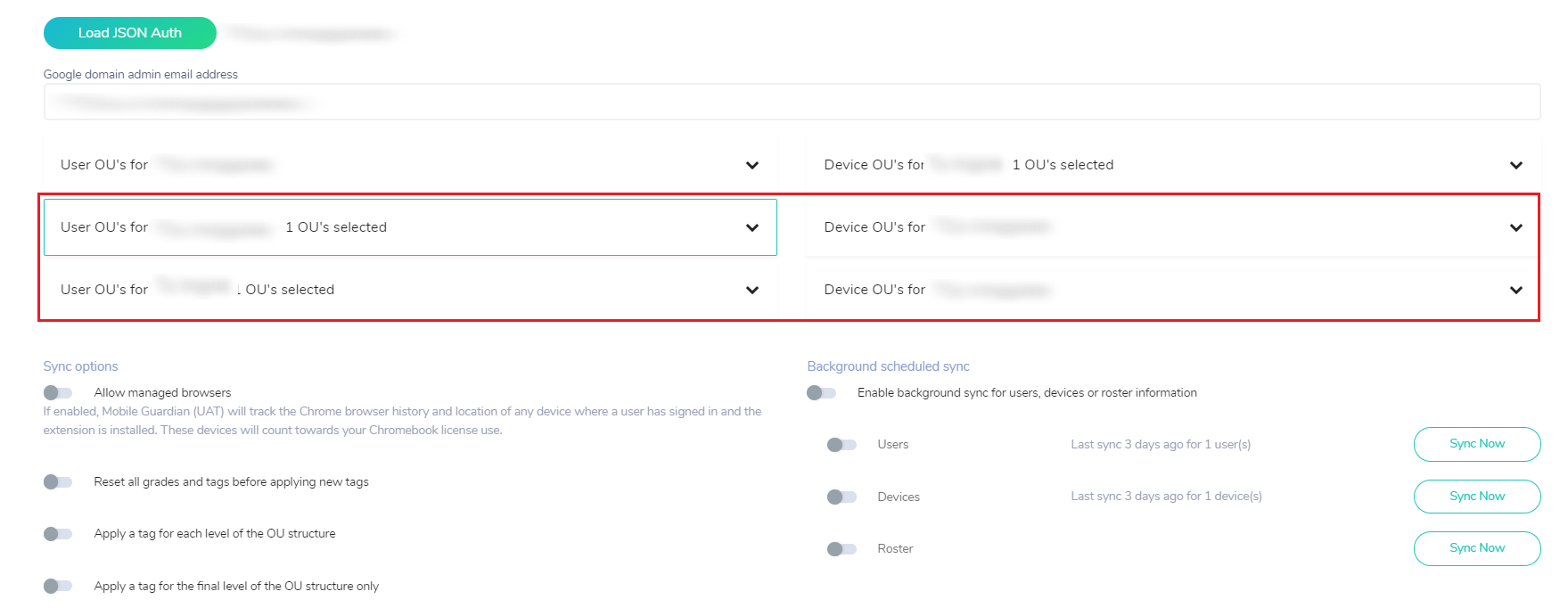**Caption:**

This is a detailed screenshot of a web page, displaying several UI elements and options. At the top left corner, there is a green pill-shaped bar, adjacent to which certain elements have been intentionally blurred out. Beneath this region, there is a partially blurred box, followed by the text "User OU's for," which is also blurred and accompanied by a down arrow. Similarly, "Device OU's for" is followed by the text "one OU selected" and a down arrow.

Below this, a box with a red outline appears, containing four lines of text. On the left side, both lines state "User OU's for," with portions blanked out and having one OU selected with a black down arrow. This specific box has a blue outline around it. On the right side, both lines mention "Device OU's for," with further information being blanked out and including down arrows.

Further down, there are sync options presented. Four options are listed on the left, while the right side shows "Background Scheduled Sync," though neither has selected options. All toggles are gray. The sync options listed include:
1. Allow Managed Browsers
2. Reset of Grades and Tags Before Applying New Tags
3. Apply a Tag for Each Level of the OU
4. Apply a Tag for the Full Level of the OU Only 

Under the "Background Scheduled Sync" section, there are various options for enabling background sync for users, devices, and other information, with specifics for routers. Each of these categories on the right side includes blue pill-shaped buttons labeled "Sync Now," none of which have been selected.